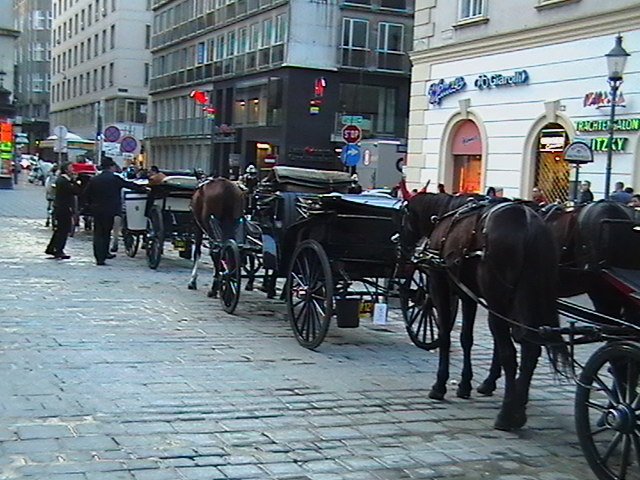This is a digital photograph capturing a street parade in an urban setting, featuring old-fashioned carriages drawn by horses. The scene is set on a paved street with gray cobblestones, some of which shine with patches of wet areas. Four brown horses with long black tails and manes are visible, adorned with leather tack and straps. These horses are pulling carriages that are black and brown, with one carriage having a distinctive white seat and large round spoked wheels. The procession is moving diagonally from the lower right to the upper left of the image. On the left side, several men are seen tending to the carriages.

The cityscape in the background showcases a mix of architectural styles. Starting from the upper left to the upper right, there are tall buildings ranging from very old gray structures to newer designs. One notable building features lighter gray on top and black at the bottom with numerous windows, while another has a faux brick upper section in very light gray and a bright white bottom with blue and yellow signage in an unreadable foreign language. The buildings have arched doorways and multiple windows, further highlighting the urban environment. The street scene is bustling with activity, with people standing around and attending to the carriages.